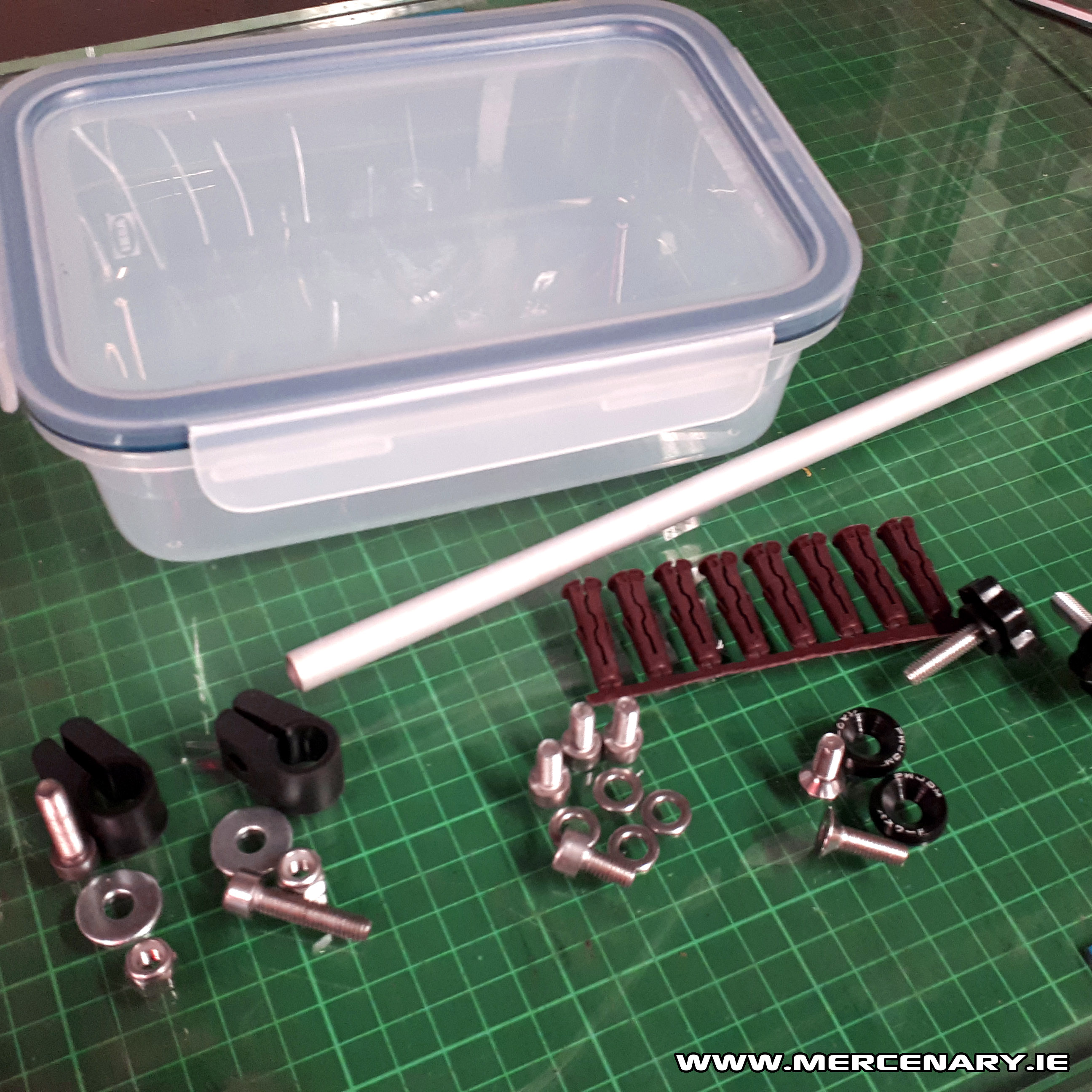This color indoor photograph captures a detailed scene on a green gridded mat, likely inside a manufacturing facility or business. Centered around the image is an arrangement of various hardware and plastic components. An elongated, empty white plastic Tupperware container with snapping lid flaps, prominently sits in the upper left region of the photo. Nearby, extending toward the foreground, is a white plastic rod or tube. Scattered across the bottom of the image are an assortment of screws, bolts, nuts, washers, and black rings, all sorted into small piles. These components appear to be for assembling some mechanical or structural item. Notably, the green mat features lighter green grid lines forming squares, which might be used for measurement or placement guides. At the lower right-hand corner, a text line reads, "www.mercenary.ie."